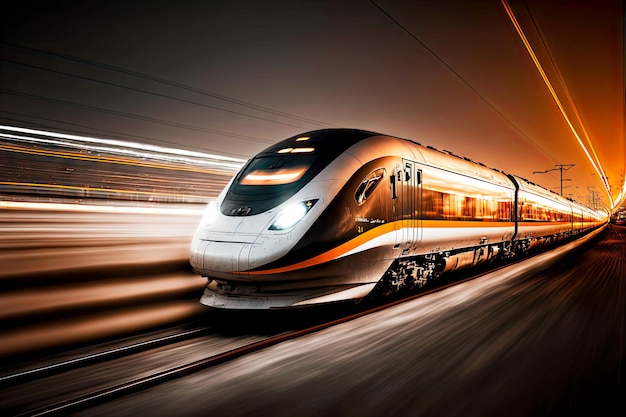The image captures a high-speed bullet train racing towards the viewer at night, embodying an idealized portrayal of modern transportation. The sleek train, which has a distinctive bullet-shaped front with a curving nose, is primarily black with accents of silver and orange. It is moving at such a velocity that the surroundings blur into streaks of color—silver, white, yellow, and orange—particularly to the front left side of the train. The power lines and telephone poles in the dark, nighttime sky add a sense of perspective and depth. The train itself is a marvel of design, with a black top and sides adorned with orange and white trim, giving it an ultra-modern and dynamic appearance. The ground beneath is barely visible, shrouded in a blurry haze of motion, while the pale brownish-gray environment adds to the overall nocturnal ambiance. The sky holds an intriguing hue of deep orange towards the upper background, further emphasizing the sense of speed and the train's cutting-edge design. The train appears to have five or six cars, each contributing to its streamlined, elongated form as it glides along double tracks, with no human presence visible in the image.